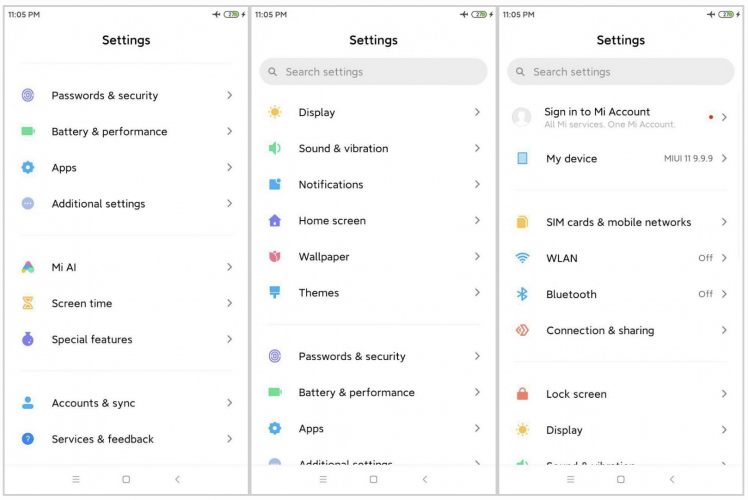The image showcases three smartphones displayed side-by-side, each presenting their settings menu. Each screen is framed by a thin grey lining, and all are shown against a white background. The time on all three screens reads 11:05 p.m., and in the top-right corner, the battery percentage icon is visible.

### Left Screen:
This screen does not feature a search bar at the top. It is divided into three primary sections:
1. **Passwords and Security**
2. **Battery and Performance**
3. **Apps**
4. **Additional Settings**
   
Following are:
1. **MIAI**
2. **Screen Time**
3. **Special Features**
   
Lastly, the section includes:
1. **Accounts and Sync**
2. **Services and Feedback**

### Middle Screen:
This screen includes a search bar at the top. The categories listed are:
1. **Display**
2. **Sound and Vibration**
3. **Notifications**
4. **Home Screen**
5. **Wallpaper**
6. **Themes**
   
Next, it continues with:
1. **Passwords and Security**
2. **Battery and Performance**
3. **Apps**
   
The fourth category here is cut off, making its name unreadable.

### Right Screen:
This screen, also featuring a search bar at the top, lists the following categories:
1. **Sign into MI Account**
2. **My Device**
3. **SIM Cards and Mobile Networks**
4. **WLAN**
5. **Bluetooth**
6. **Connections and Sharing**
   
Lastly:
1. **Lock Screen**
2. **Display**
   
The third option at the bottom here is also cut off and unreadable.

At the bottom of each screen, there are three icons, color-coded in grey, indicating navigation buttons or menu tabs. All text on the screens is in black, making it easily readable against the white background.